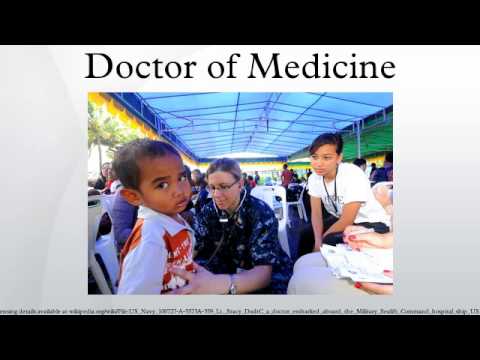The image depicts a scene from a medical camp featuring a nurse with a stethoscope, centrally positioned, examining a young boy wearing a collared white and orange (or red) shirt. The boy, who has a darker complexion and short black hair, appears somewhat worried and is looking directly at the camera. To the right of the nurse, a young woman with tied-up black hair and wearing a white shirt is seated, observing the interaction. The setting is under a blue awning or covering, which is prominently visible at the top of the image. Surrounding the photograph is a light grey background with black strips at the top and bottom. Above the photograph, the words "Doctor of Medicine" are written in black lettering.